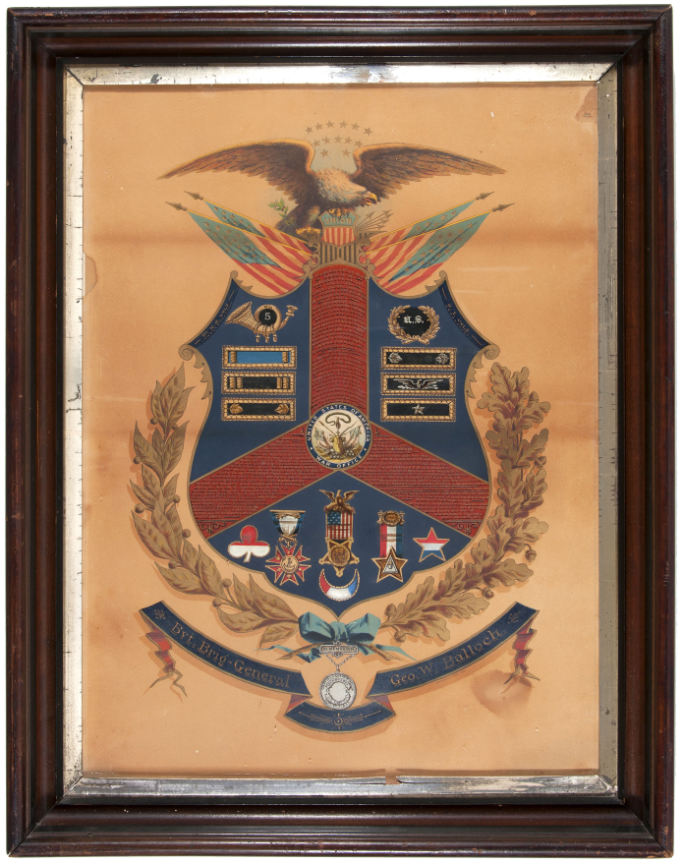This full-color photograph captures a meticulously crafted display featuring a coat of arms. The piece is encased in a dark, rich wooden frame with a simple, understated design, suggesting it has been carefully stained. Inside the main frame, there is a lighter-colored wooden border that complements the scene. The background is a natural, unstained brown wood, revealing a few grainy areas that add a touch of rustic texture.

Central to the display is a highly decorative, patriotic painting dominated by military themes. An impressive winged eagle with outstretched wings soars at the top, epitomizing vigilance and strength. Below the eagle, a complex coat of arms includes elements evocative of the American flag, with multiple flags and military insignia intricately incorporated into the design. The primary colors of the coat of arms are blue and red, symbolizing valor and perseverance. Despite some small, unreadable text at the bottom, the display passionately conveys a sense of national pride and military honor.